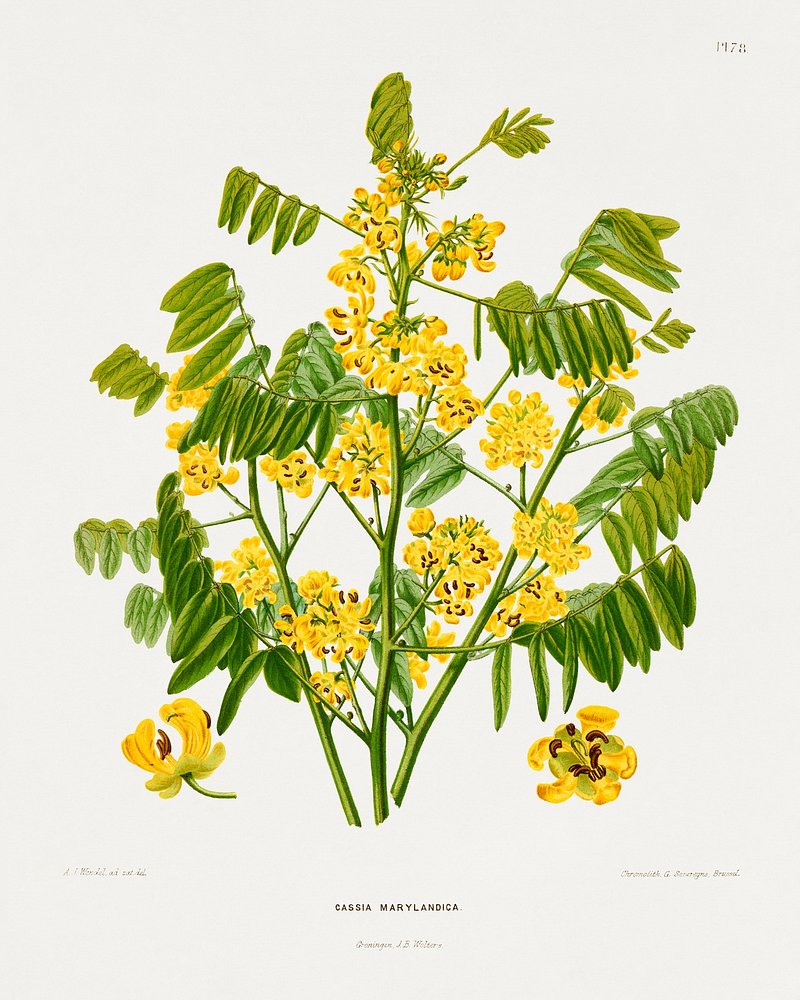The image is a detailed color drawing of a Cassia marylandica plant, rendered on a light gray piece of paper. The dimensions of the image are such that the left and right sides are twice as long as the top and bottom sides. The plant features a large, thick green stem with multiple smaller branches, each adorned with long, bean-shaped green leaves and vibrant yellow flowers. These flowers have yellow petals and brown filaments. A few yellow flowers have fallen off the plant, but most remain attached to the stems. On the bottom center of the image, the plant is labeled "Cassia marylandica," and additional text includes "A. Mitchell World" in the bottom left corner and "Chromoth G. Everth" in the bottom right corner. There is also text on the top right corner that reads "1473." Multiple angles of the flower are depicted, showcasing its intricate structure and natural beauty.